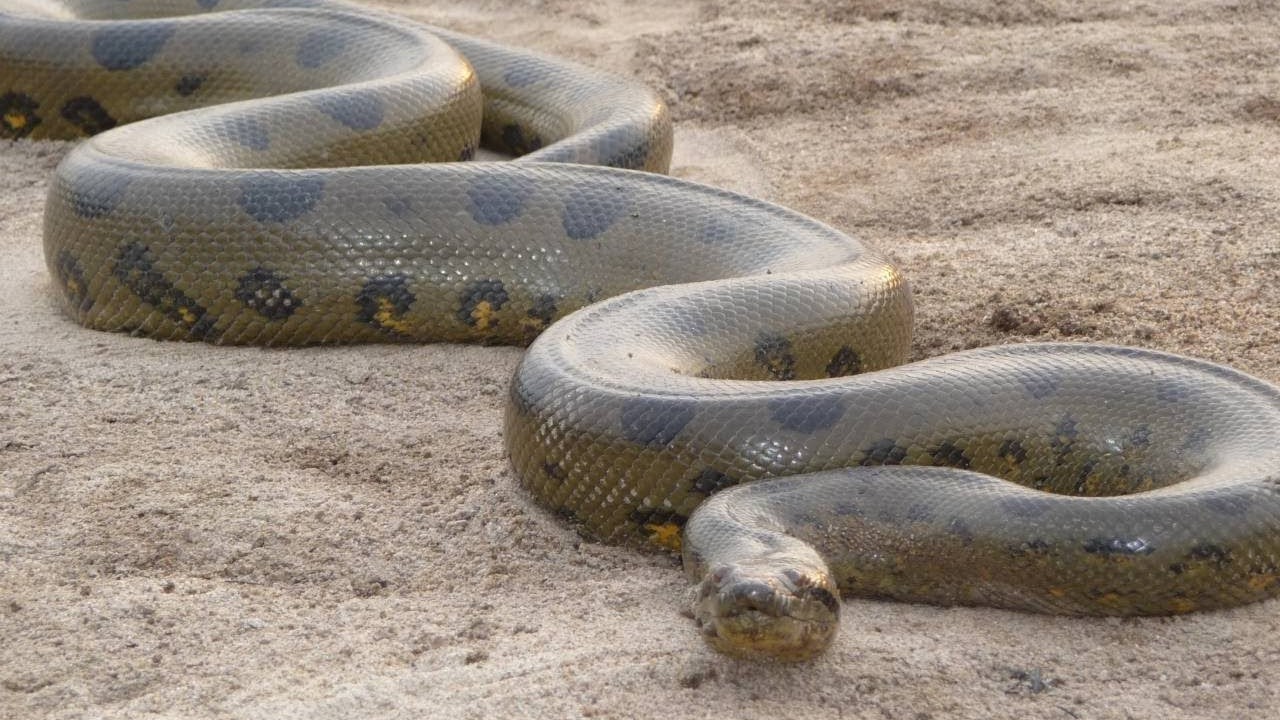The photograph captures a large snake, likely a boa constrictor or an anaconda, slithering across a sandy, arid landscape during the daytime. The snake, which appears immense and robust, displays a mix of greenish-brown hues with dark black blotches interspersed with yellow and light brown spots. Its body is sinuous, forming several S-curves, with a large midsection and a tail wrapped around towards its front. The snake’s head, comparatively small to its massive body, is oriented towards the camera, positioned slightly to the left. Shot from an overhead perspective, the image focuses solely on the snake and the surrounding sandy terrain, with no other distractions present.